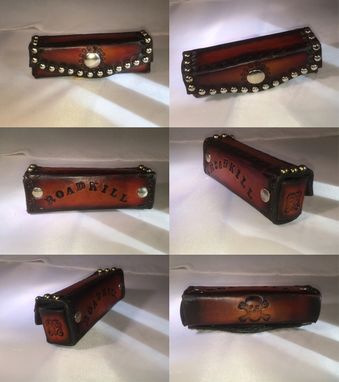This image is a grid of six photos, arranged in two pictures per row and spanning three rows, showing a small, dark brown leather pouch from various angles. The pouch, approximately the size and shape of a stick of butter or a pocketknife case, features a large steel button on its flap, which is secured with silver rivets. Notably, the flap also carries some indiscernible engraved words. The back of the pouch is engraved with the word "Roadkill," while another side displays a skull and crossbones. The images suggest the item is potentially for sale, with each photo taken under harsh lighting, creating significant shadows on the white platform on which the pouch rests.